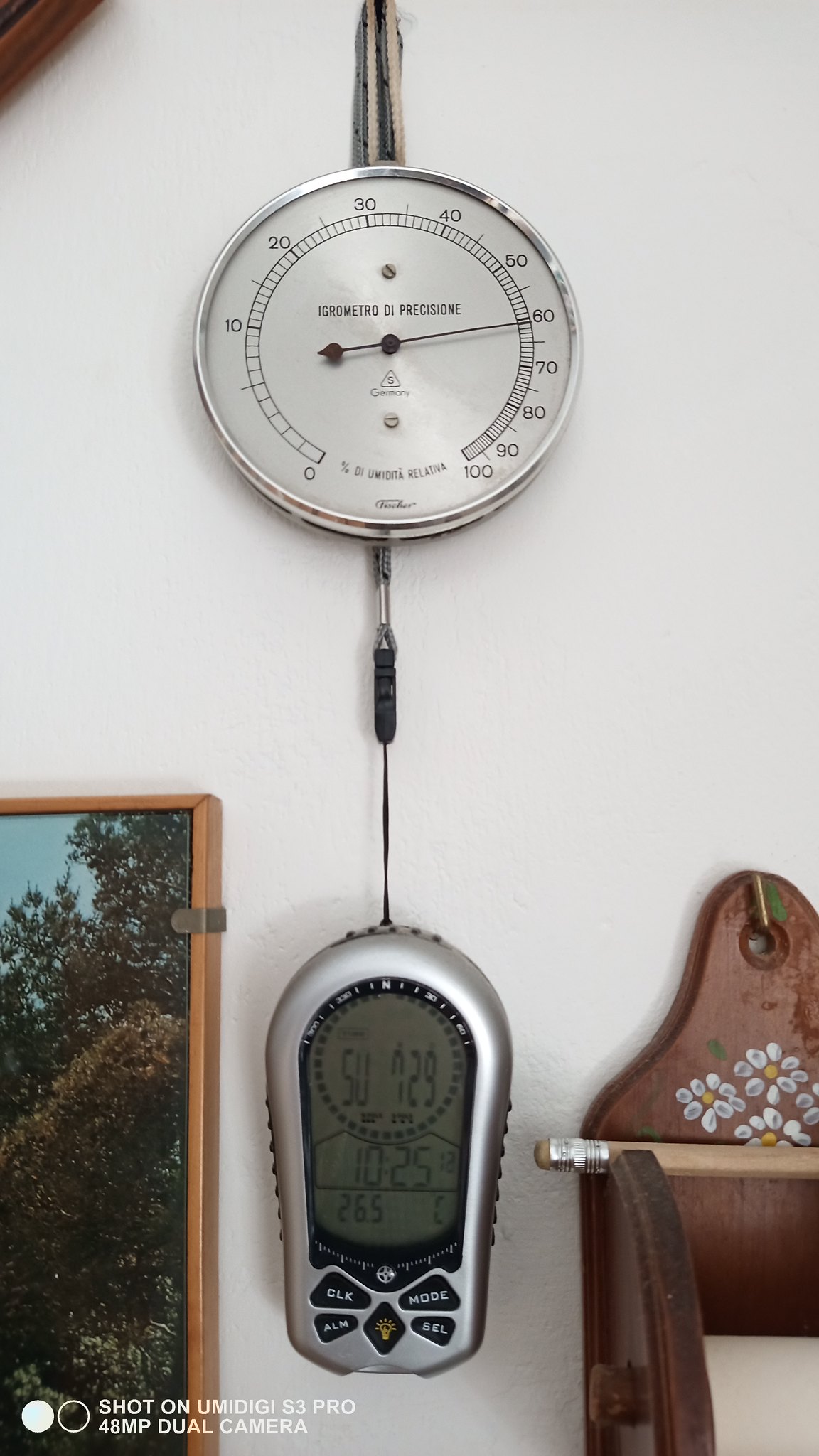This clear-colored photograph, shot on a UMIDIGI S3 Pro 48MP dual camera, captures a section of a room. The emphasis is on a white wall, where a silver circular device, possibly an analogue hygrometer or thermometer, displays numbers ranging from 0 to 100 with its hand set to around 60. The device has black font on it, including the text "Igrometro di Precisione," suggesting its Italian origin. A black wire or arm extends downwards from the device, attached to a digital reader with an LCD display showing the numbers 50729, the time 10:25 AM, and "265 C." Below this setup, towards the lower section of the photograph, is a framed painting of trees against a sky and a decorative wooden item with a pencil resting on it. The bottom left also features two white circles, one filled and one clear, next to the text indicating the camera model and its capabilities.